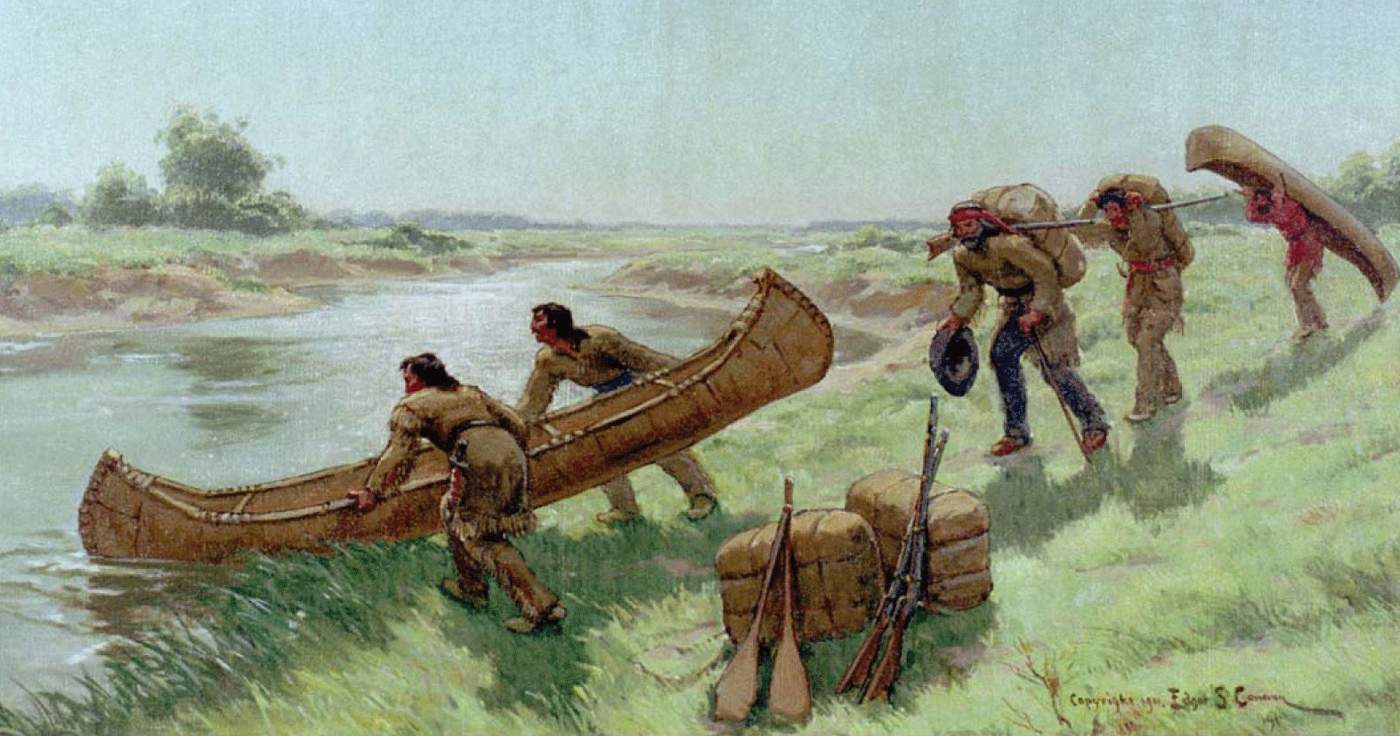This image is an old oil painting portraying a scene of Native Americans preparing to launch a canoe into a river. The artwork, possibly over a hundred years old, features five individuals with reddish dark skin, dark hair, and moccasins. They are dressed in handmade beige outfits resembling light-colored animal skins adorned with tassels. Central to the image, two of these individuals are positioning a long, light brown canoe into gray, silver-tinged water, against a backdrop of light and dark green hues cast by distant trees. 

To the right, three more individuals are descending a hillside toward the river, walking on pale green grass. The first person, with salt-and-pepper hair and a partial beard, wears light brown clothing, blue pants, and carries a rifle positioned between a large knapsack on his back and his neck. Next to him, another man with short black hair, dressed similarly, grips a knapsack around his waist with a red belt. Trailing them, a third man in a red shirt and tan pants balances another canoe on his head, supported by his arms. Near the canoe on the ground lie two light brown oars and two rifles with wooden stocks in various shades of brown and gray, propped against square hay bales.

The painting’s landscape emphasizes a lush grassy bank and a river bed with brown rocks. The sky overhead is a soft blend of faded blue with wisps of light brown. The artist's signature can be found in the bottom right corner of the painting, adding a final touch to this vivid yet subtly colored scene.